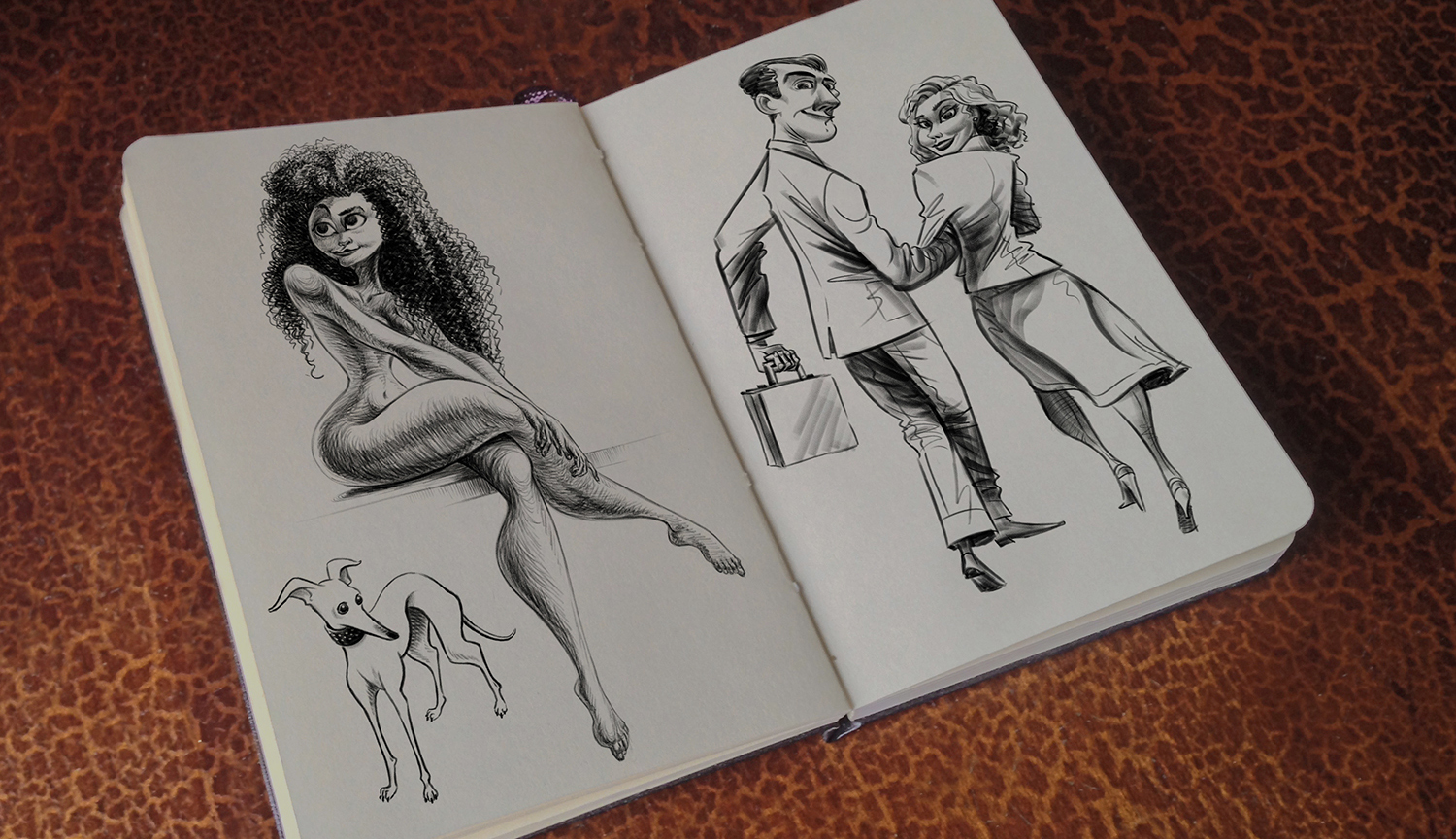The image features an open sketchbook laid diagonally on a surface resembling brown, reddish wood with a textured, giraffe-like design. The sketchbook's off-white pages display detailed pencil drawings with various characters. On the left page, there is a woman with long, curly dark hair sitting cross-legged and smiling, accompanied by a thin, poised dog. The right page depicts a well-dressed man in a suit holding a briefcase and a woman in high heels and a skirt, arm in arm, both looking back at the viewer. The book is positioned near the center of the image, though the upper right corner is slightly cut off. The setting appears to be a cozy interior, possibly someone's home or art room. The image is devoid of text and showcases a palette of browns, whites, blacks, and shades of gray.